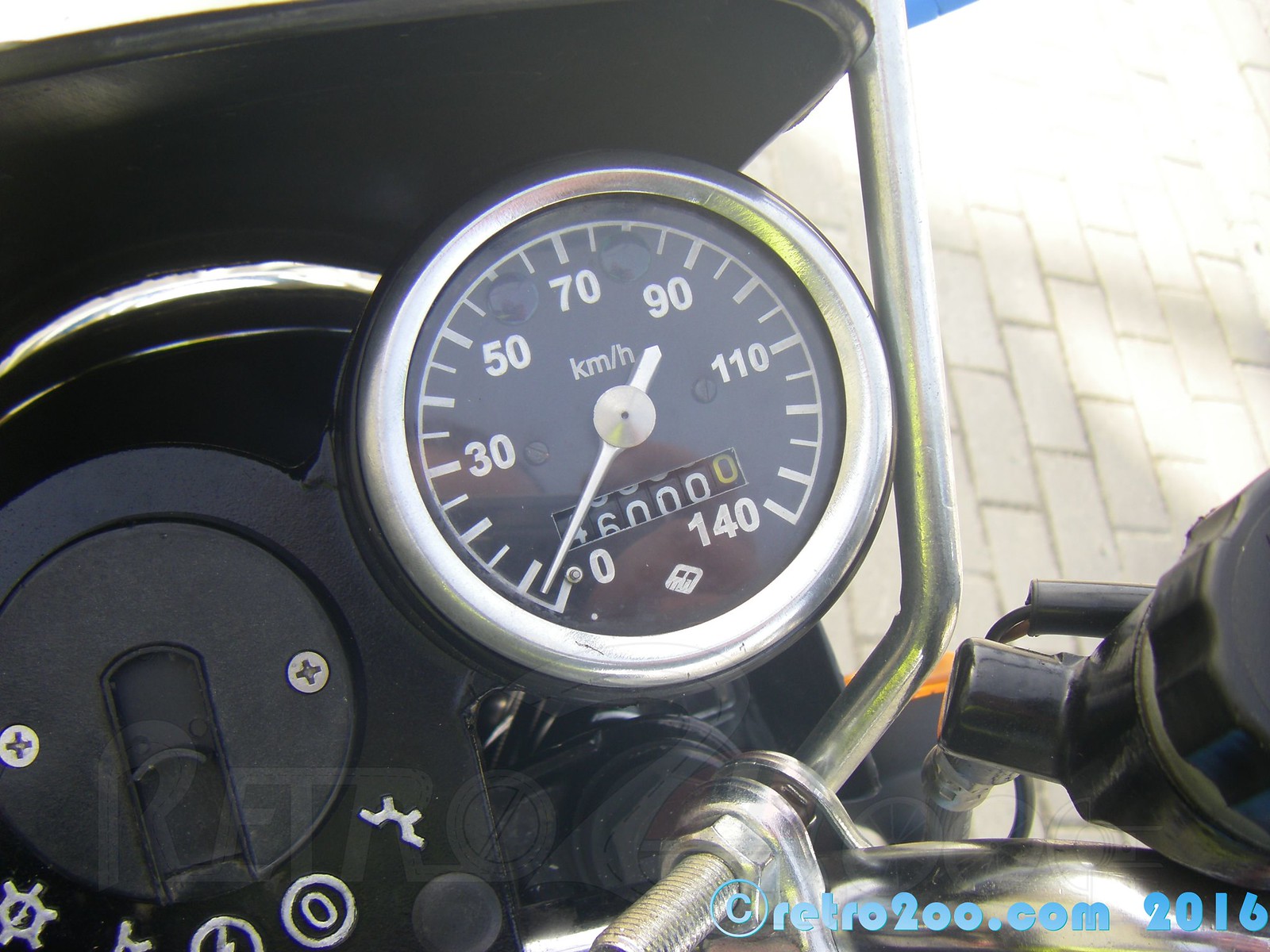This is a color photograph focusing on the dashboard of a vehicle, likely a motorbike, given the composition and elements present. The image provides a partial view of the pavement outside, located in the upper left corner, featuring vertical cream-colored rectangular bricks. The left side of the photograph is dominated by the black dashboard, which runs vertically upward. A long metal bar descends from the top about two-thirds to the right of the image, then slants diagonally towards the center.

Central to the composition is a circular speedometer with a metal rim and a brownish face, displaying white numbers: 0, 30, 50, 70, 90, 110, and 140. The silver needle points to zero. Within the speedometer's center, there is a smaller rectangular gauge with the number 16000. To the left of the speedometer, a black wheel with two silver bolts is visible.

In the bottom right-hand corner, overlay text in light blue reads "@retro@200.com 2016." Additionally, there are various symbols at the bottom of the dashboard, including round shapes and one that resembles half of a gear. A full gear icon is located on the left, and a curved white line appears at the top of the black surface of the dashboard. This meticulously detailed photograph captures the intricate elements of the motorbike's dashboard, blending mechanical precision with visual clarity.